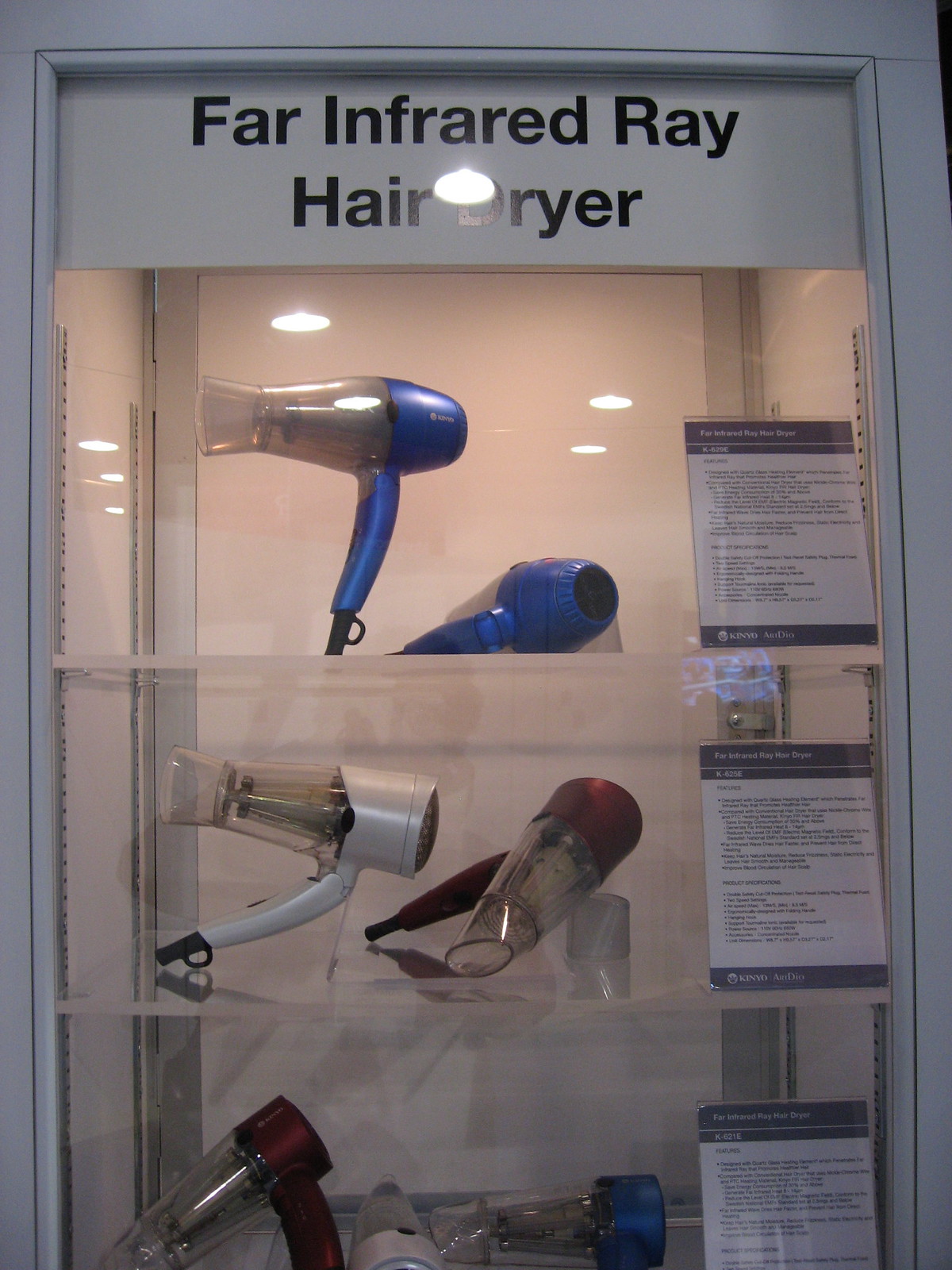The image depicts a display case showcasing Far Infrared Ray Hair Dryers, as indicated by the black lettering on a white background at the top of the case. The display cabinet has a glass front, reflecting ceiling lights, which slightly obscures some details. The case contains three clear shelves, although the bottom shelf is partially cropped out in the frame. 

On the top shelf, there is a blue hair dryer accompanied by a sign detailing its features. The second shelf holds two handheld hair dryers, one silver and grey, and one red, both with accompanying descriptive signs. The lowest shelf, though partially out of frame, reveals a red hair dryer that is propped up, a white one laying down, and a blue hair dryer, all with description pages. This arrangement suggests a store or booth environment where the products are likely for sale, each clearly labeled to highlight their specifications and models.